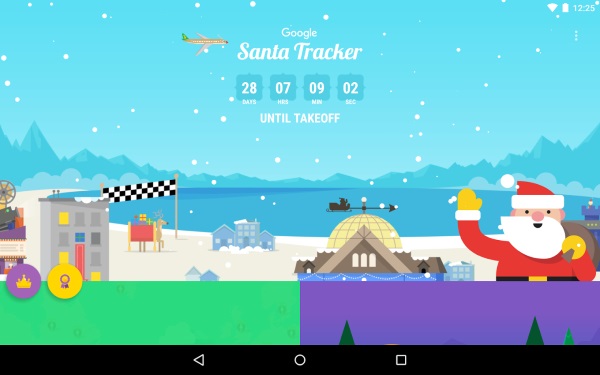The image depicts a festive Google webpage themed for the holiday season, specifically for tracking Santa Claus. At the top, the header reads "Google Santa Tracker" prominently. Just below this header, there is a countdown timer indicating "28 days, 7 hours, 9 minutes, and 2 seconds until takeoff," adding to the excitement of the holiday season.

The vibrant and colorful webpage background showcases a scenic nature setting with an ocean, and Santa Claus, dressed in his classic red suit with a white beard and yellow gloves, cheerfully waves at the viewers. Snowflakes gently fall across the scene, enhancing the festive atmosphere.

To the right of the ocean, a gray building is visible, flanked by patches of green and purple, resembling Christmas trees and other holiday decorations. At the top right corner of the image, essential UI icons such as Wi-Fi and battery status are shown.

At the bottom of the screen, a navigation bar features a back arrow, a white circle, and a white square on a black background, implying a mobile or tablet interface. A checkered flag and a reindeer pulling a sleigh filled with gifts are also part of the festive scene, reinforcing the holiday spirit and the purpose of tracking Santa's journey. Overall, the page exudes a celebratory mood, perfect for the holidays.